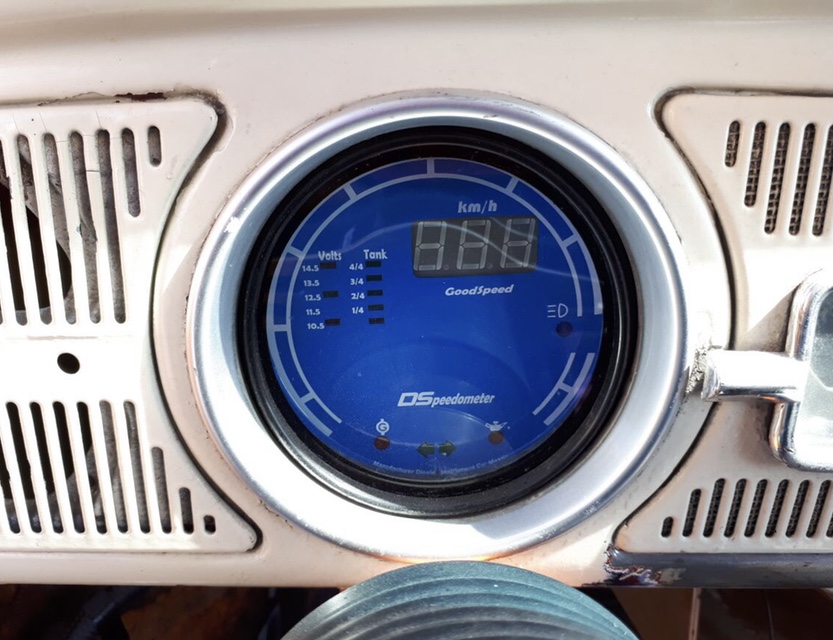Indoor color close-up photograph of a digital speedometer installed in a vintage dashboard, likely from a car or moped from the late 1950s. The dashboard features a classic metal look, flanked on either side by evenly spaced vertical grille slots. At the center, where the original instrument cluster would have been, there is a chrome bezel. Within this bezel, the speedometer has been upgraded to a digital unit with a blue face.

On the left side of the digital display, there are two columns of indicators. The first column is labeled "Volts" at the top, followed by a series of letters and black horizontal squares. The second column is labeled "Tank" with five black rectangles below it, each corresponding to fractional fuel levels of four-fourths, three-fourths, two-fourths, and one-fourth.

The right upper portion of the display houses the speedometer itself, a three-digit LED display that is currently not illuminated. Above the speedometer, white lettering reads "KM/H," and below it, "Good Speed" is inscribed. The lower center portion of the display is labeled "DS" or "D Speedometer."

In the foreground, part of the green semi-circular steering column is visible, adding to the vintage aesthetic of the setup.